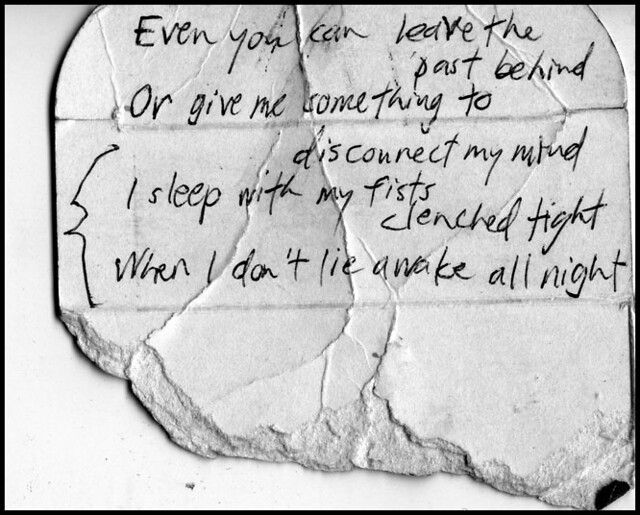The image depicts a scanned or photographed piece of paper or possibly a broken tile wall. A large square image with a black border framing the entire piece. The background is a cracked, light gray material resembling stone, with visible creases and wrinkles, especially around the bottom left corner. The primary focus is an inspirational quote, handwritten in black ink, that reads:

"Even you can leave the past behind or give me something to disconnect my mind. I sleep with my fists clenched tight when I don't lie awake all night."

The text spans approximately six lines from the top to the middle of the image. Additionally, there is a squiggly bracket-like line on the left side of the last two lines of the quote, adding emphasis. The overall texture and appearance of the image, combined with the quote, evoke a sense of juxtaposition between the fragile, cracked background and the profound message inscribed upon it.